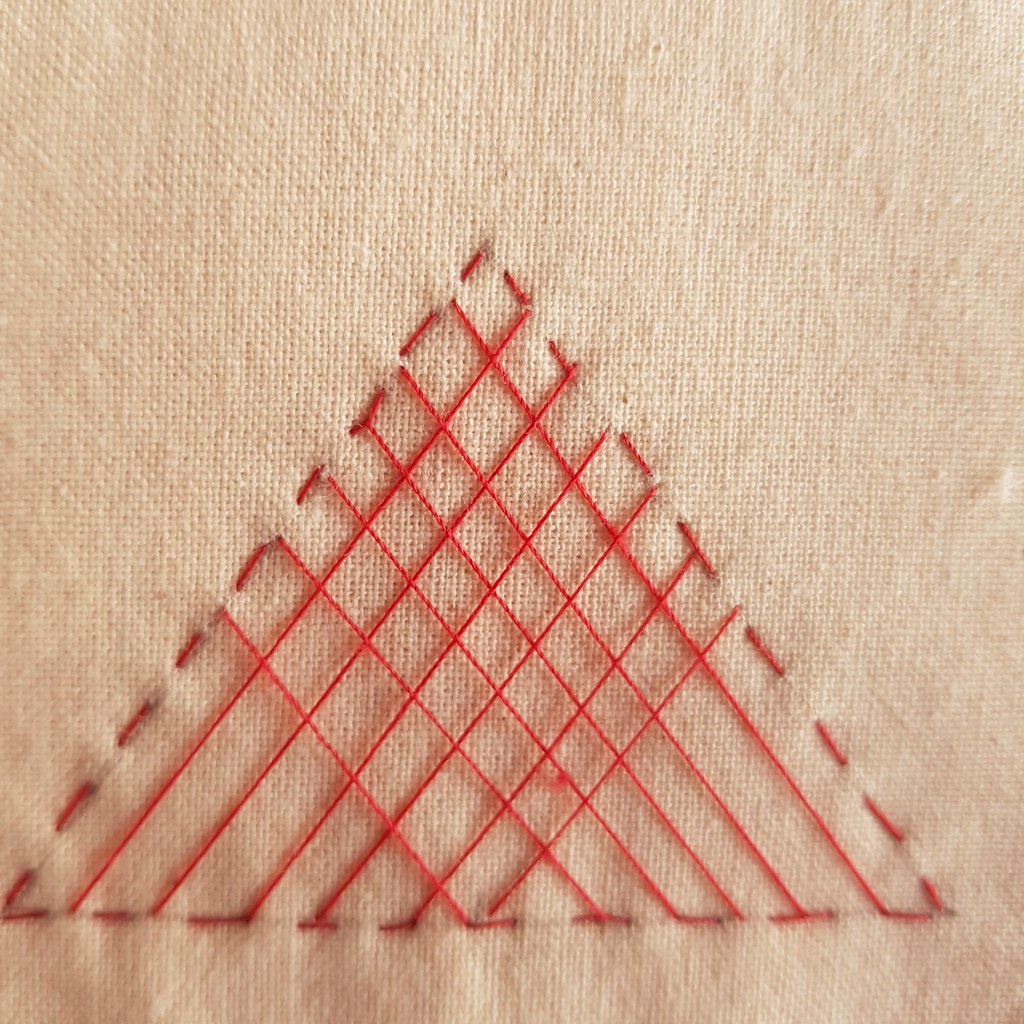The image features a rectangular piece of tightly knit fabric, possibly made of materials such as cotton, burlap, canvas, or linen, with a light beige or wheat color. The fabric serves as a background for an intricate and partially completed red cross-stitch embroidery. The main embroidered pattern is an upward-pointing triangle with a dotted outline created by spaced stitches. Within the triangle, red threads crisscross diagonally, forming a series of rhombus or diamond shapes. The lines run from the top left to the bottom right, and from the top right to the bottom left, creating a detailed and decorative criss-cross effect. The work is only half-finished, indicating that the person embroidering still has more to complete.